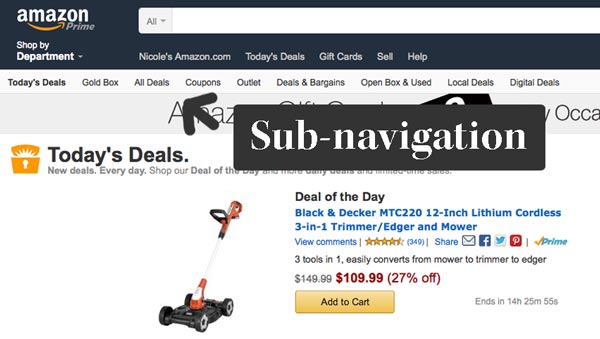This left-to-right horizontal image captures a typical browsing session on Amazon, specifically showing a section of the webpage dedicated to deals. The interface suggests that it can be accessed via the Amazon app or through their website on a computer or smart device. 

At the very top of the image, there's a black navigation bar featuring the Amazon Prime logo, a "Shop by Department" dropdown, and the word "All" in gray, indicating the selection of all departments. Adjacent to these elements is a white search bar currently devoid of any input.

Directly below this, the webpage highlights various navigation links in white text, including "NicolesAmazon.com," "Today's Deals," "Gift Cards," "Sell," and "Help." Following this, the background of the webpage shifts to a lighter gray tone, prominently displaying the "Today's Deals" section. This section is bolded for emphasis and includes various subcategories such as "Gold Box," "All Deals" (marked by an arrow for easy navigation), "Coupons," "Outlet," "Deals and Bargains," "Open Box and Used," "Local Deals," and "Digital Deals."

A gray box featuring another arrow pointing towards "All Deals" includes the text "Sub Navigation" in bold white letters, indicating additional navigational options. Below this, the primary content area displays a prominent orange icon that reads "Today's Deals," accompanied by the phrases "New deals every day" and "Shop our Deal of the Day," though part of the message is obscured by the sub-navigation box.

The image specifically includes a snapshot of a product listing for a Black and Decker three-in-one Trimmer Edger Mower. The product details shown include the star rating, number of reviews, price, and an add-to-cart button, providing users with essential information at a glance.

Overall, the image offers a comprehensive glimpse into the organized and user-friendly layout typical of Amazon's shopping interface, emphasizing the extensive deals and easy navigation options available to its users.